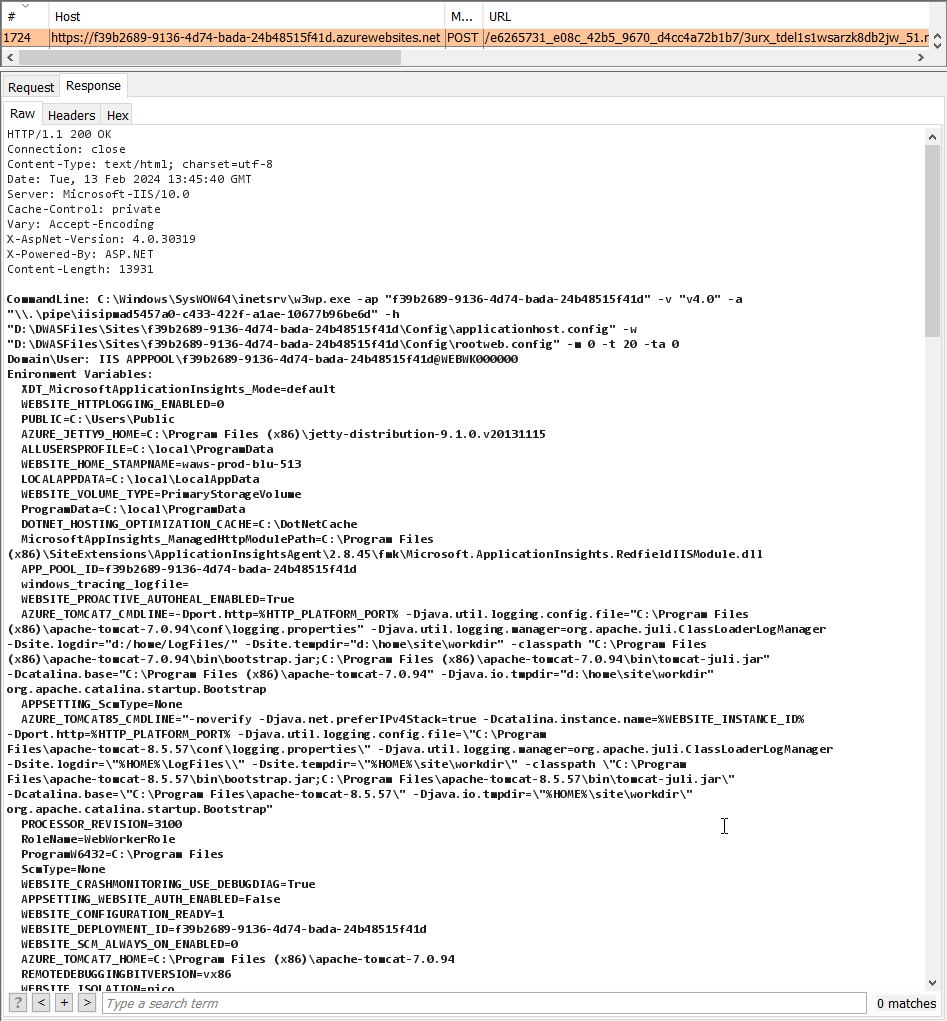The image depicts a detailed webpage displaying lines of code. At the very top, there is a thin, pink horizontal bar running from left to right, which contains the web address formatted as a random string of numbers, dashes, and other indistinguishable characters. Above this bar, there is a small text label reading "Host." Directly beneath the bar, "Request Response" is prominently displayed.

The code itself begins immediately below, with headers and values such as "Connection: close," "Content-Type," "Date," "Server," "Cache-Control," "X-AspNet-Version: 4.0," "X-Powered-By," and "Content-Length: 13931." The majority of the document is filled with what appears to be gibberish to the untrained eye—an assortment of random words, letters, numbers, and symbols typical of a coded web document. The text throughout the page is small, black, and uniformly styled, extending consistently from the top to the bottom of the page.